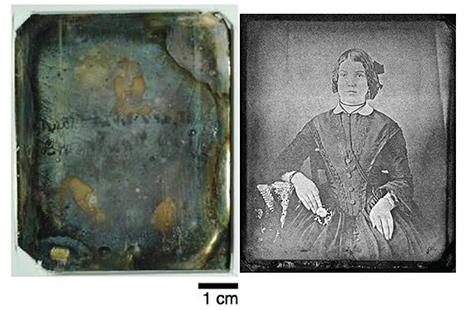The restored image ensemble includes two side-by-side photographs of a woman, with slight variations in details and dimensions. The left photo displays significant damage, resembling an artifact affected by fire, leaving the image singed and the woman's figure almost indiscernible. Aged and with muted colors transitioning from grayish-blue to orange and brown, it appears to have dark green and brown edges, further indicating its deterioration. In contrast, the right photo, meticulously restored to grayscale, features the same woman sitting down with a serious expression. She is depicted in a period dress, her hair styled up, with her hands resting in her lap. The restoration precision highlights her torso and part of her dress, preserving the vintage essence against a plain, grayish background. Both images are similarly sized, roughly five to six centimeters in height, as indicated by a one-centimeter scale beneath them. The restored photo is encased in a black outer frame, devoid of additional text or figures.